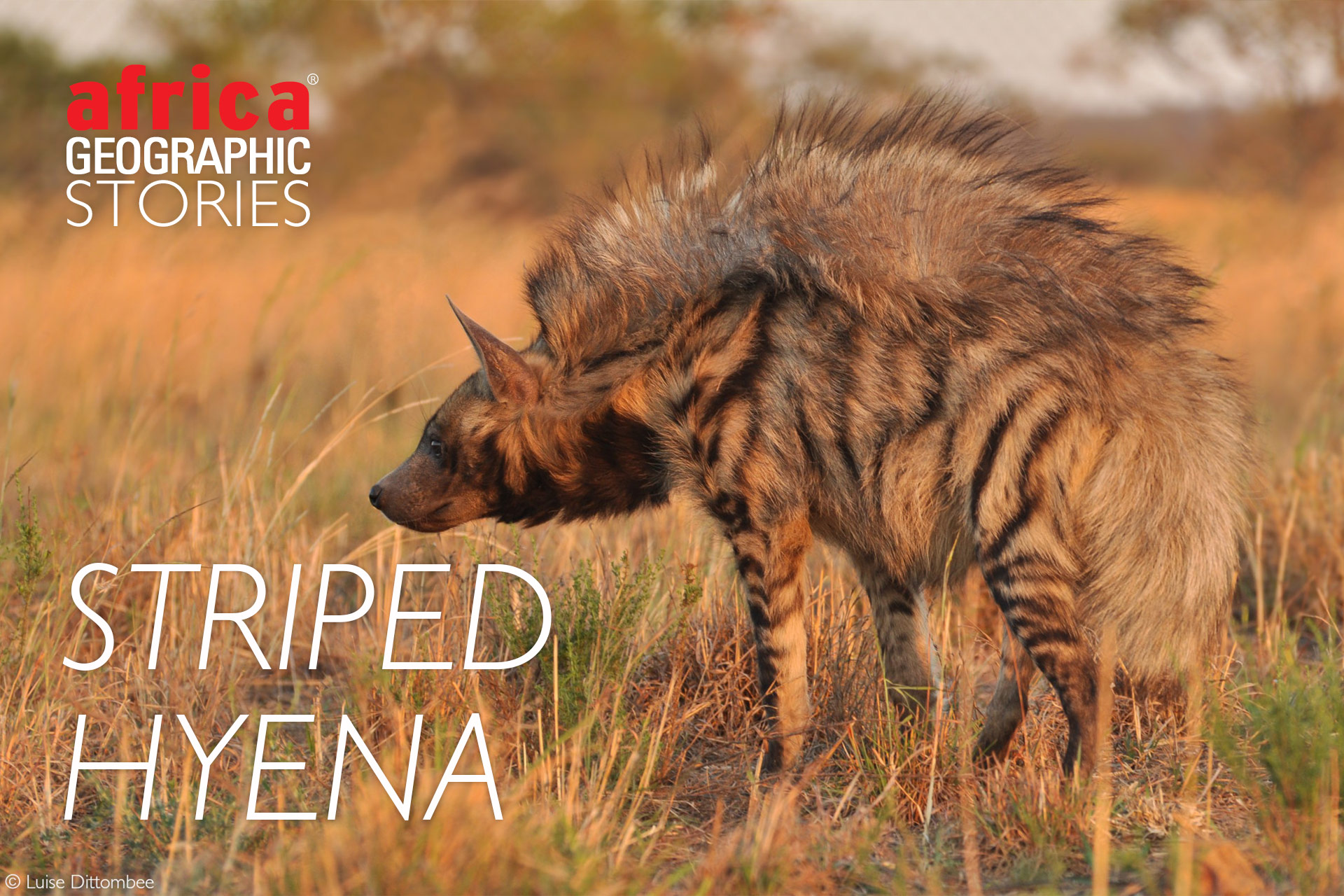The image features a striped hyena with distinctive light brown and black fur, creating a striking contrast along its body. The hyena's fur on its back appears choppy and spiky, standing up prominently along its spine. It has a sleepy look in its eyes, and its head is turned to the left, with its tail to the right. The hyena is positioned among tall, yellowish, and light brown dehydrated grass, with some patches of green visible. The background includes blurred trees and a bit of sky at the top. In the upper left corner of the image, red text reads "Africa" and larger white text underneath states "Geographic Stories". Below this, in white text, the image is titled "Striped Hyena". Additionally, the lower left corner contains a small circle with a "C" and the name "Luis de Tambi".